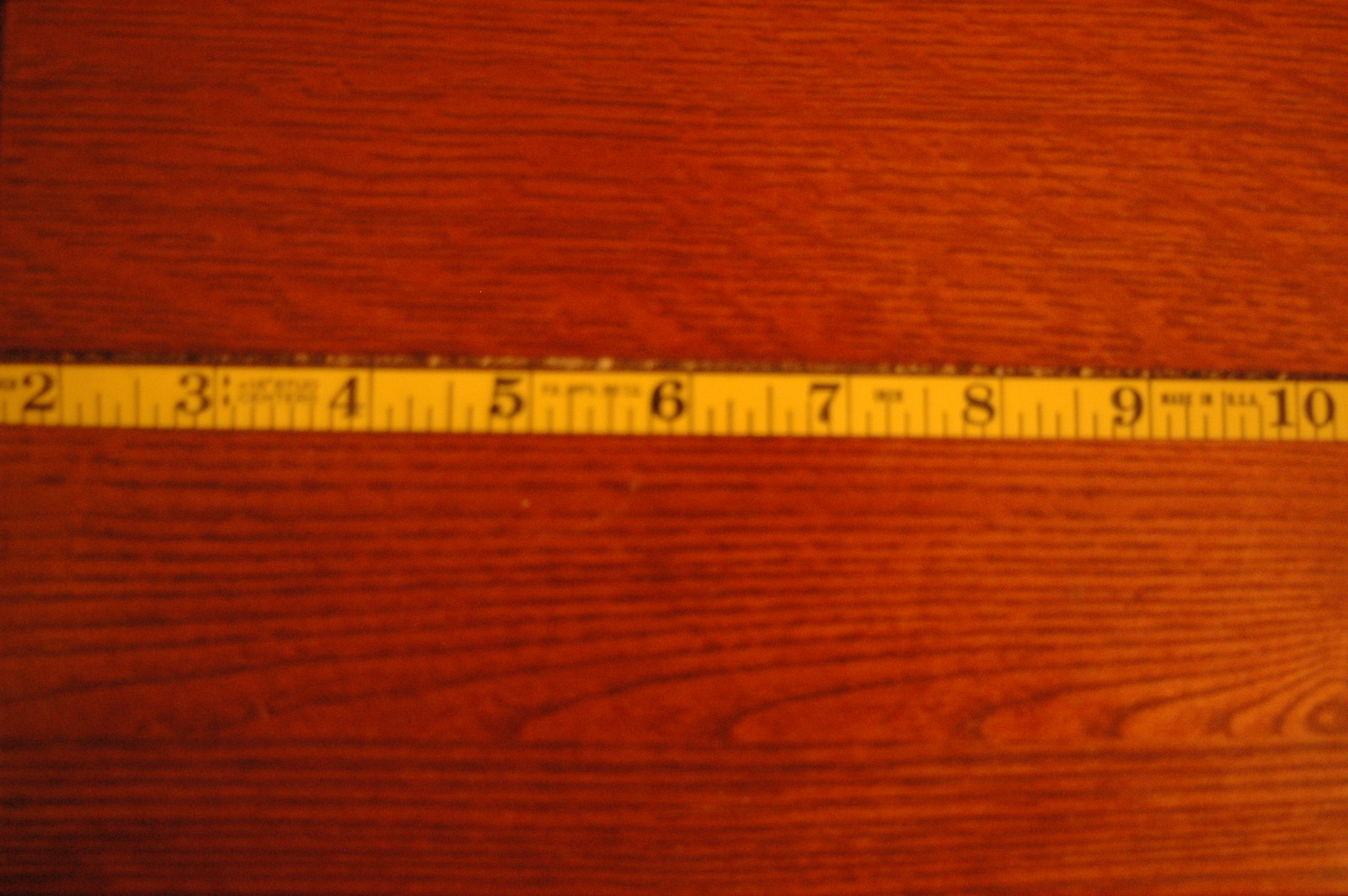The image features a reddish-brown wooden surface, possibly a table or platform, spanning the entire background. Centrally placed and running horizontally across the middle of the image is a bright yellow measuring tape. The measuring tape, starting a little before the number 2 and extending slightly past the number 10, is marked in centimeters. Each numeric marking—2 through 10—is displayed in black, accompanied by corresponding black lines for precise measurement. The tape, slightly out of focus at the ends, is bordered by a thin black line along its top edge. A bit of light is cast onto the tape, enhancing its visibility against the wooden background.